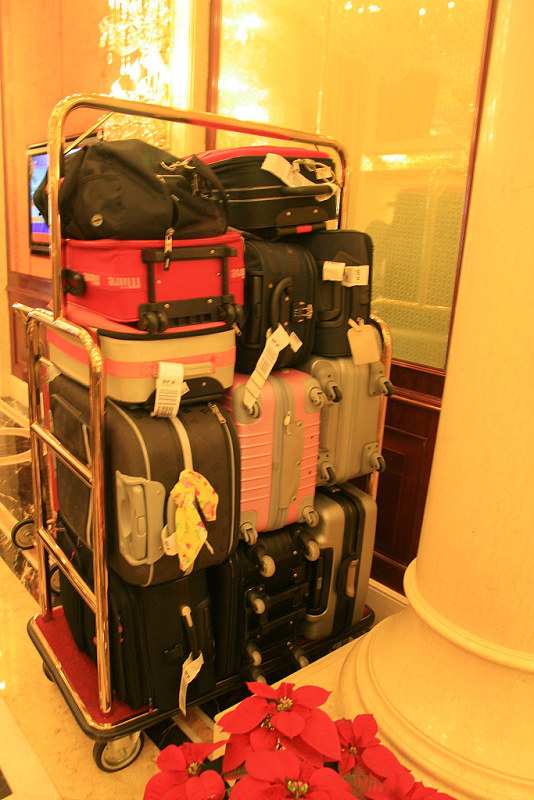This photograph, likely taken with a cell phone, captures a hotel luggage trolley laden with approximately twelve suitcases of various colors, including black, gray, pink, and red, many adorned with luggage tags or identifiers. The trolley, with its sturdy brass stanchions and wheels, features a red carpet base and tall bars suitable for hanging clothing. It occupies about two-thirds of the image towards the left. The hotel lobby's warm lighting casts an orange glow over the scene. Directly in front of the trolley stands a large white pillar adorned with a poinsettia plant at its base. The background reveals white lights and a TV mounted on the wall above a wooden panel, with a glass panel adjacent to the trolley, potentially serving as a window.